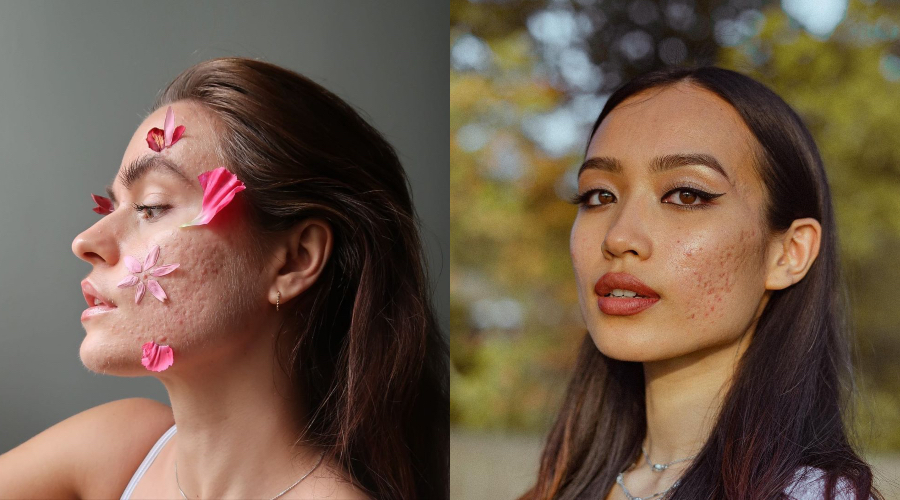This image is a side-by-side comparison of two women, highlighting their unique beauty and shared features. The woman on the left has auburn hair swept back, light skin adorned with pink flower petals, and is captured in profile looking slightly downward against a gray background. She wears light orangish-pink lipstick, sports pronounced darker eyebrows, large eyelashes, and has brownish eyes. Notably, she has pockmarks from acne scars on her cheeks but exudes a distinct beauty. The woman on the right, set against a blurred background with green trees, has long brownish hair and is looking directly at the camera with her head slightly rotated to the right. She has coffee-brown eyes, dark eyeliner, full dark eyebrows, and deep peach-colored lipstick. Like the woman on the left, she bears acne scars on her cheeks. She also wears a double silver chain necklace and appears to be of Asian descent. Both women, possibly in their late 20s or early 30s, are beautifully styled to celebrate their skin conditions and natural beauty.